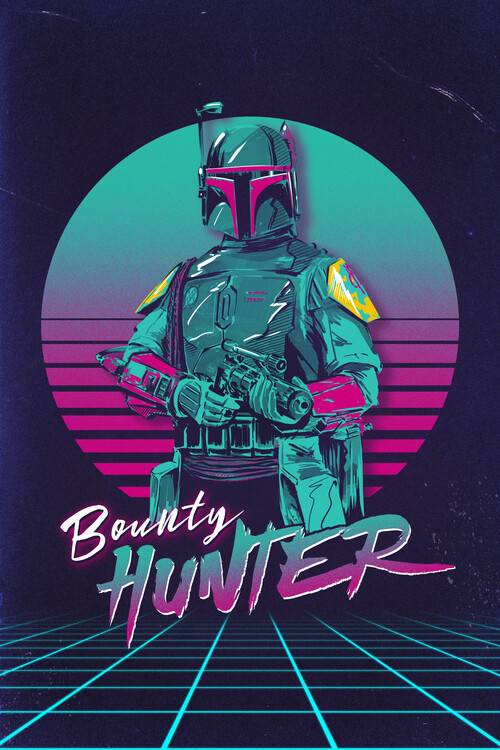The promotional artwork, likely for a movie poster titled "Bounty Hunter," showcases a highly stylized and futuristic design. At the center, a figure—a bounty hunter clad in full futuristic hunting gear—stands defiantly with a gun raised. The design pays homage to 80s aesthetics with a vibrant color palette featuring black, white, various shades of blue, pink, yellow, purple, and gray. The bounty hunter’s armor includes distinct aqua blue highlights, yellow shoulders, and pink accents on the mask and forearms, with the gun also hued in blue. 

Behind the figure is a circular emblem that transitions from aqua blue at the top to darker pink at the bottom, segmented by lines. This circular motif is set against a dark blue background that evokes a space-like vibe. Below the bounty hunter is a tiled floor, depicted in a grid pattern with small squares, reminiscent of a mason-style grid.

The only text on the image reads "Bounty Hunter," with 'Bounty' rendered in white cursive letters and 'Hunter' in bold blue and pink uppercase letters. The overall composition is highly artistic and professional, suggesting a promotional piece likely intended for a sci-fi or action movie.